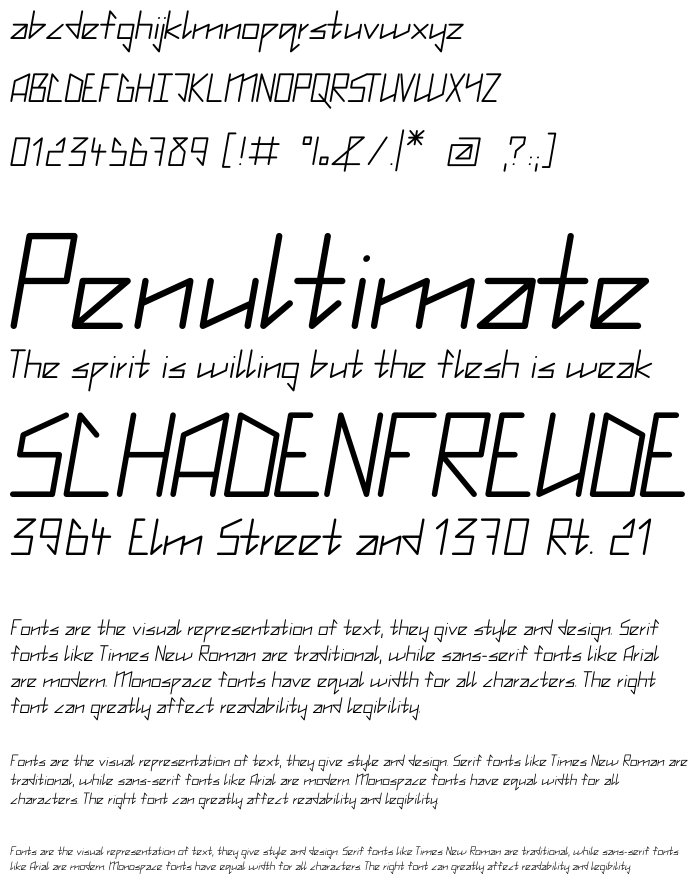This vertical rectangular image features a white background with no outside border and showcases a variety of text in different fonts. At the top, there are lines displaying the alphabet in both uppercase and lowercase letters, followed by the numbers 0 to 9 and a selection of special characters including a parenthesis, exclamation point, pound sign, percentage symbol, forward slash, asterisk, and question mark. Below these characters, in large black typography, is the word "penultimate." Underneath this, in a cursive style, appears the phrase "the spirit is willing but the flesh is weak." Next, in the same large black letters but in all capitals, is the word "SCHADENFREUDE." Following this, in smaller text, the addresses "3964 Elm Street" and "1370 Route 21" are listed. The image also contains a couple of paragraphs about fonts and their impact on readability and legibility, which get progressively smaller in size towards the bottom.